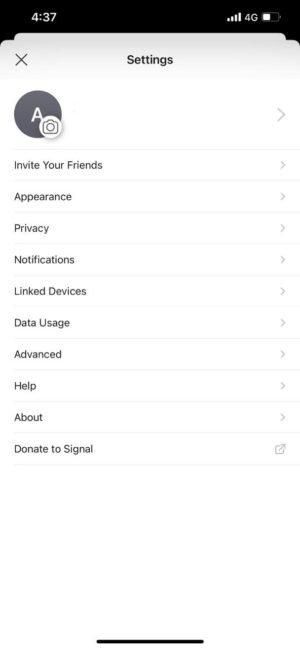The screenshot displays the settings menu of the Signal app. At the very top, the status bar shows it's 4:37, with full bars of 4G service and a battery level at approximately 56%. The settings menu itself appears as a white pop-up box with an 'X' on the left to close it. 

Titled "Settings," this section includes a gray circle with a white 'A' at the center serving as the user's profile picture. There is a small white camera icon in a circle at the corner of this profile picture, allowing users to change it.

The menu options listed within the settings are:

1. Invite Your Friends
2. Appearance
3. Privacy
4. Notifications
5. Linked Devices
6. Data Usage
7. Advanced
8. Help
9. About
10. Donate to Signal

Each of these options, except for "Donate to Signal," has a small arrow on the right side, indicating that clicking them will expand the menu. The "Donate to Signal" option features a square with an arrow pointing outwards, indicating it will redirect the user to an external website.

The interface is primarily white with black text, and there is a small black bar along the bottom of the screen. The status information at the very top is placed on a black background.